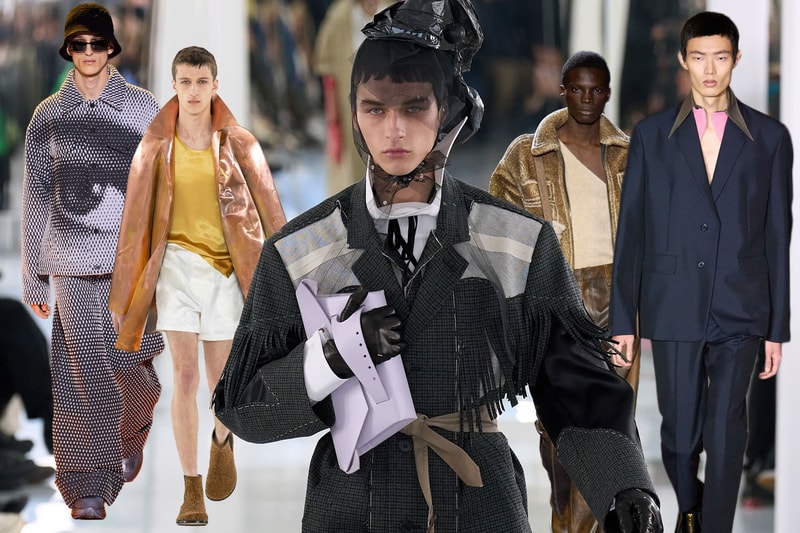The central figure in this fashion photo is striking in their avant-garde ensemble. They stand out prominently, dressed in a black outfit that exudes a blend of mystery and theatricality. The character wears a crumpled black hat, accentuated by netting that covers their face and is carefully tied in a bow under the chin. Complementing this enigmatic look is a hairdo featuring uneven bangs that frame their stoic expression. Their top, crafted from what appears to be canvas material, is adorned with fringes, adding texture to their attire. Black gloves cover their hands; one hand elegantly clasps a white case against their body, while the other hangs naturally by their side. Adding a subtle touch of color, a brown belt cinches their waist.

In the background, four distinct figures contribute to the eclectic atmosphere. On the far left, one individual wears a gray suit adorned with an eyeball graphic, paired with a matching gray bucket hat. Next to them, a person stands out in a yellow shirt, white shorts, brown shoes, and an orange coat, providing a vivid pop of color. Further to the right, a Black man dons a luxurious brown velvet coat over a white shirt with an asymmetrical cut, combined with matching velvet pants. The ensemble is completed by an Asian man on the far right, who wears a dark blue suit set off by a pink button-up shirt and tie, finished with an exaggeratedly pointed large collar. Collectively, the group presents an intriguing mix of fashion-forward styles, each unique in their own right yet harmoniously contributing to the overall composition.